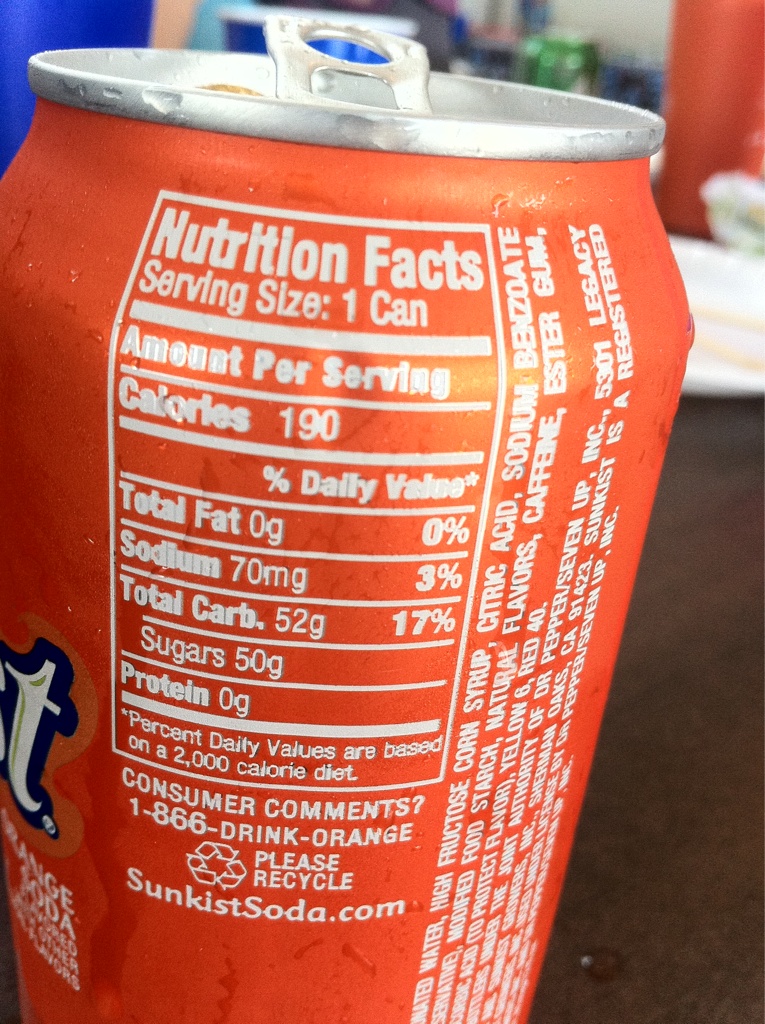The image depicts an orange Sunkist soda can prominently featuring the brand's iconic design. The cylindrical aluminum can, equipped with a standard pop-top, boasts vibrant orange coloring indicative of its citrus-flavored content. The nutritional facts are prominently displayed on one side of the can. They indicate that a single serving (one can) contains 190 calories, 0 grams of fat, 70 milligrams of sodium, 52 grams of total carbohydrates (including 50 grams of sugars), and 0 grams of protein. These values are based on a 2,000 calorie daily diet. 

Additionally, consumer information includes a toll-free number for comments and a reminder to recycle. The can also lists the manufacturer's website, sunkistsoda.com, for further information. The ingredients are clearly spelled out towards the bottom, ensuring transparency for the consumer. This detailed label provides all essential information while reflecting the refreshing and zesty essence of the Sunkist brand.